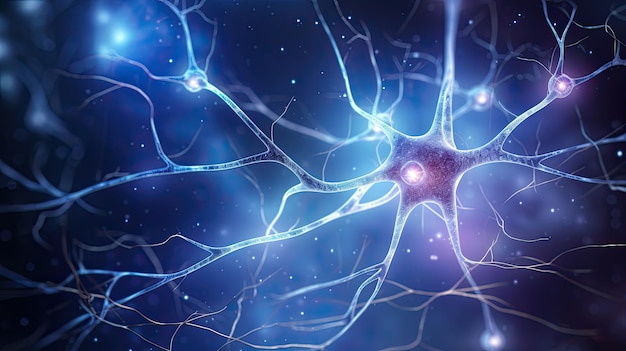The image is a computer-generated rendering of a nerve synapse with a dark background peppered with white specks, suggestive of a microscopic view of neural connections. Dominating the scene slightly to the right of center is a star-shaped, purplish-black synapse with tendrils extending from it like roots or lightning bolts. These tendrils exhibit a gradient of colors, ranging from a glowing bluish-white to darker shades of black, purple, and pink. Each tendril connects to other similar synapses scattered throughout the composition, each one housing a glowing ball of light at its core. The vibrant colors and intricate details, including the long nerve strands and glowing cells, contribute to the image's overall clarity. This highly detailed and artistic 3D depiction presents an imaginative view of neural connections, highlighted by blue and purple hues amidst a predominantly dark setting.